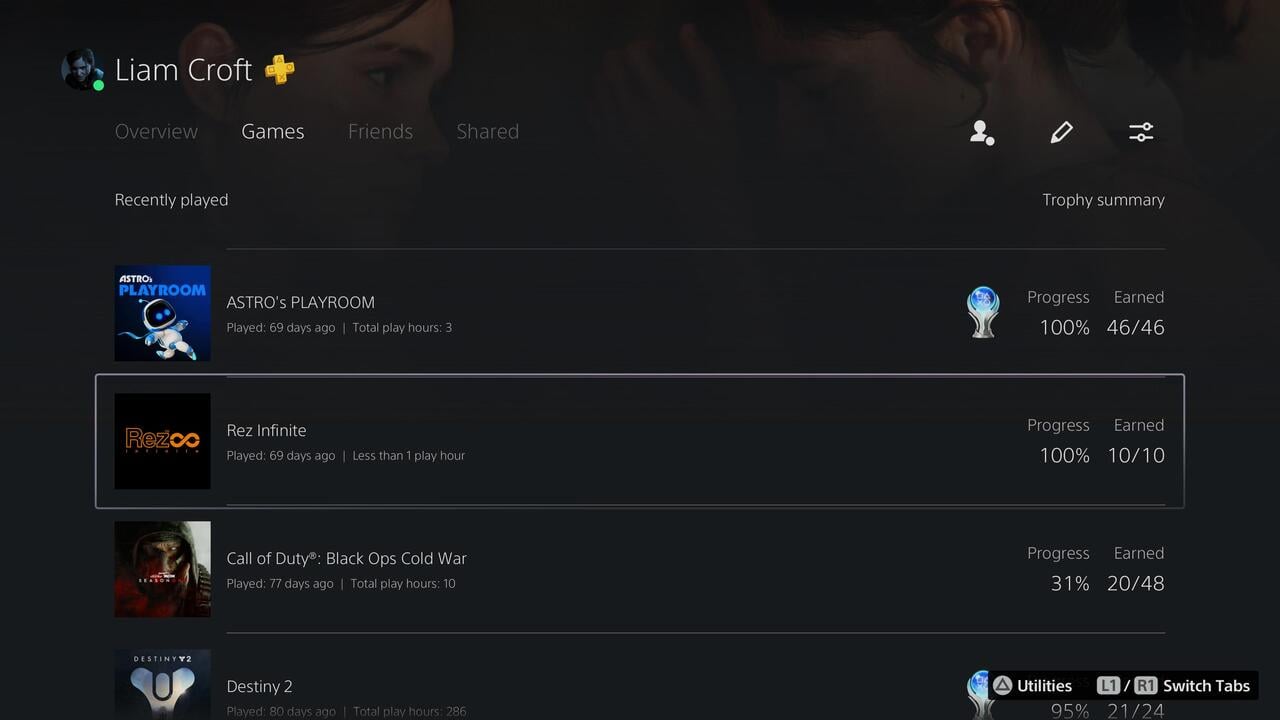A screenshot of a gaming profile from a gaming website, displayed on a horizontal rectangular frame with a black background. 

### Header Contents:
- **Top-Left:** A small circular avatar of a man with a green dot indicating online status.
- **Next to Avatar:** The user's name, "Liam Croft," in white text, followed by an orange plus sign.
  
### Navigation Bar:
- **Left to Right:**
  - "Overview" in dark gray.
  - "Games" highlighted in white.
  - "Friends" in dark gray.
  - "Shared" in dark gray.
  - A gray icon resembling a person with a white dot.
  - A gray pencil icon.
  - A gray filter toggle button.

### Main Content:
- **First Section:**
  - **Top-Left:** "Recently Played" in light gray.
  - **Top-Right:** "Trophy Summary" in gray.
  - **Game Entry 1:**
    - **Thumbnail:** Cartoon astronaut.
    - **Title:** "Astro's Playroom" in gray. Repeated to the right of the thumbnail.
    - **Details:** "Played 69 days ago" and "Total play hours: 3" in gray.
    - **Right:** An icon of a globe indicating progress, "Progress: 100%" and "Earned: 46/46" in gray.
  
- **Second Section:**
  - **Game Entry 2:**
    - **Thumbnail:** Blank black image with "Res" and an infinity symbol in orange.
    - **Title:** "Rez Infinite" in gray.
    - **Details:** "Played 69 days ago," "Less than one hour played" in darker gray.
    - **Right:** "Progress: 100%" and "Earned: 10/10" in gray.
  
- **Third Section:**
  - **Game Entry 3:**
    - **Thumbnail:** Hooded person.
    - **Title:** "Call of Duty: Black Ops Cold War" in light gray.
    - **Details:** "Played 77 days ago," "Total play hours: 10" in darker gray.
    - **Right:** "Progress: 31%" and "Earned: 20/48" in gray.
  
- **Fourth Section:**
  - **Game Entry 4:** (Partially visible)
    - **Thumbnail:** A 'V' shape.
    - **Title:** "Destiny 2" in light gray.
    - **Details:** "Played 50 days ago," "Total play hours: 286."
    - **Foreground Information:** A circle with a triangle inside labeled "Utility" and a prompt "L1/R1 switch tabs."

### Interface Guide:
At the bottom-right, icons and instructions for switching tabs using L1 and R1 buttons are visible.